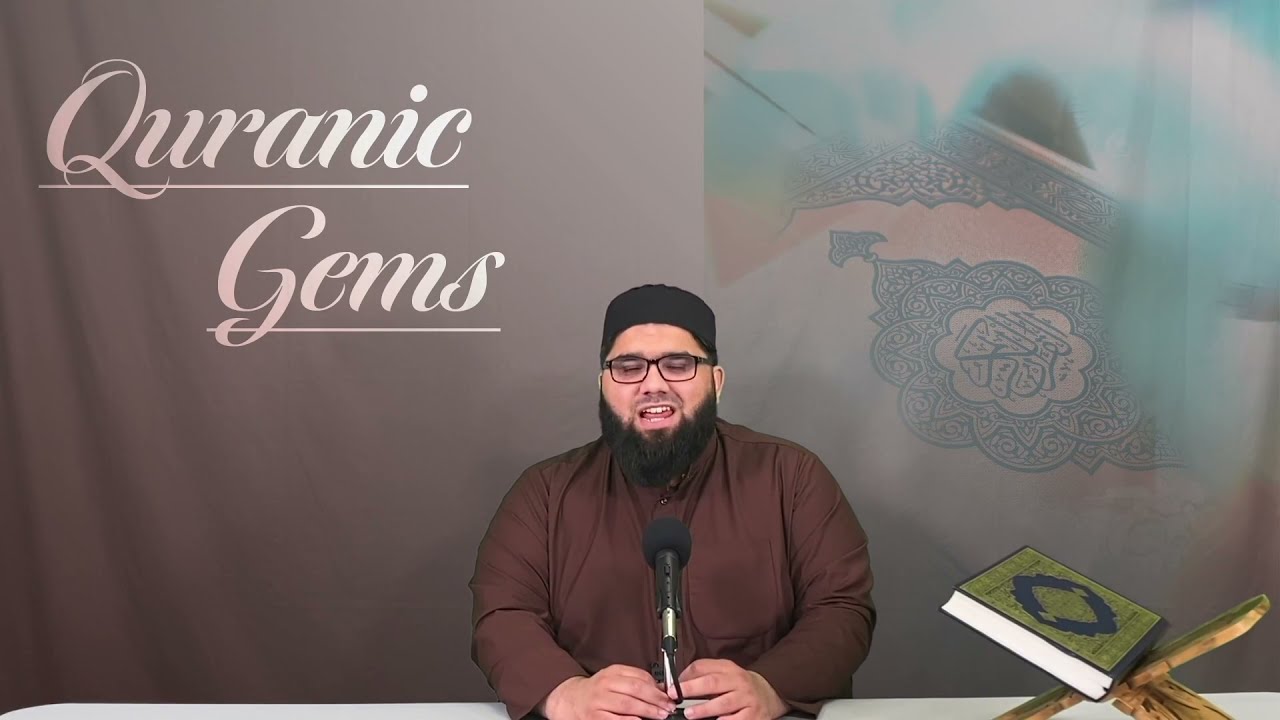The image depicts a man of likely Middle Eastern descent, dressed in a long-sleeved brown robe, seated at a table with a microphone. He wears a black, brimless, cylindrical hat that appears to be of religious significance and sports black reading glasses. He has a distinctive black beard that comes to a tip, with only a faint outline of a mustache. The man is positioned centrally, facing forward, with his eyes closed and mouth open, indicating he is speaking. His hands are clasped around the base of the microphone, which is mounted on a stand. Behind him is a brown curtain featuring the words "Quranic Gems" in ornate script, underlined in both instances. To the right of the man, there is a fanned-out bookstand holding what is likely a Quran with a green cover and a blue circular design. The upper right portion of the background shows a somewhat floral pattern, adding a decorative element to the scene. This detailed setup suggests a formal or religious podcast or discussion setup.